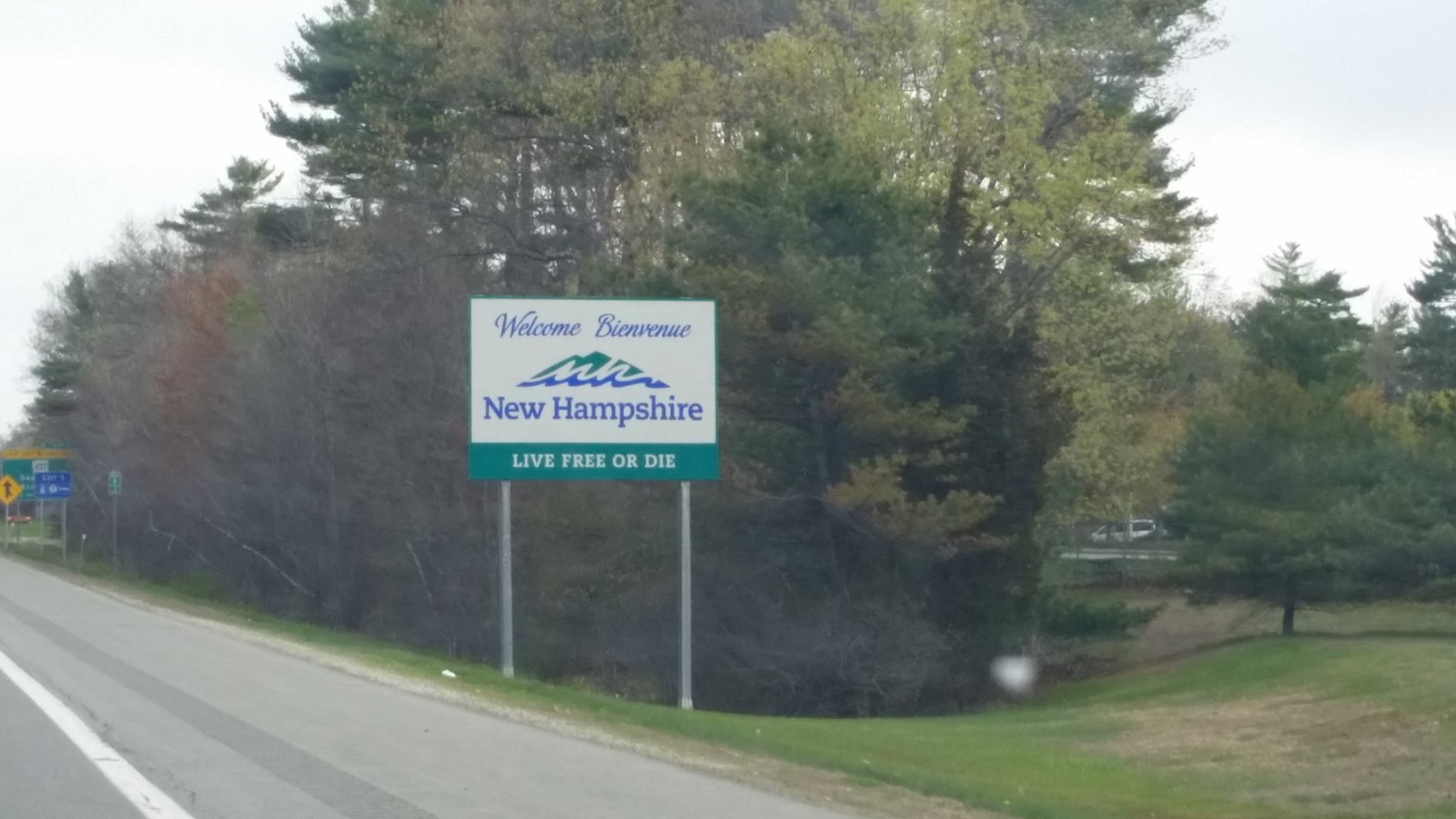This photograph, apparently taken from a moving vehicle, captures a welcoming sign along a smooth, pale grey highway in New Hampshire. In the bottom left corner, the flat asphalt road features a white line marking the shoulder, adjacent to a dark grey rumble strip. Dominating the center-left of the frame is a prominent state sign, white with a teal outline. The sign greets visitors with "Welcome, Bienvenue, New Hampshire" in blue text. Below this, a green and blue stylized mountain bears the initials "NH." The state's motto, "Live Free or Die," is inscribed on a teal background at the sign's base. Background elements include a grassy hillside and a dense array of trees – mixing green pines, a large green deciduous tree, and numerous bare deciduous trees in muted brown and grey hues. Additionally, a cluster of indistinct, multi-colored signs appears near the road on the left. The sky overhead transitions from a pale blue to white, adding a serene backdrop to the scene.